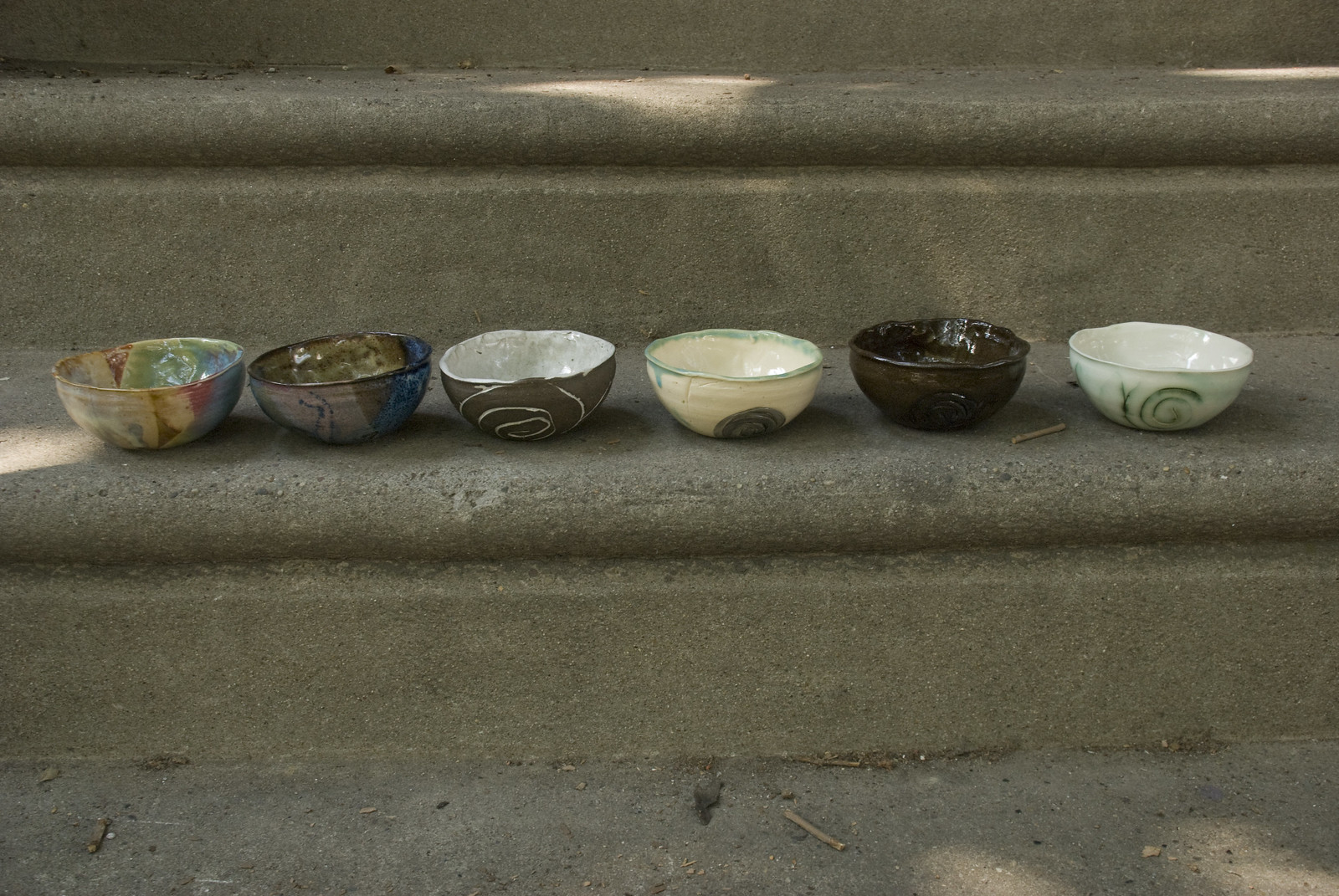In this image, six ceramic bowls of varying colors and patterns are aligned on a thick concrete step. A second concrete step is visible behind them, with sunlight gently illuminating areas of both steps, particularly the middle upper step and the left section of the lower step where the bowls rest. Each bowl, likely handmade, showcases unique designs and finishes, hinting at pottery class origins with a subtle shine in their middles and slightly scalloped, uneven tops.

From left to right: the first bowl is a vibrant collage of dull yellow, red, green, and blue. The second bowl features a dark palette with colors like dark blue, black, dark brown, and a purplish hue. Next is a bowl that evokes a coconut theme, brown with possible white lines on the outside and completely white inside. The fourth bowl is cream-colored with a mint green rim. The fifth bowl is a solid dark brown. The last bowl boasts a white exterior adorned with green snails and a swirly green line pattern, while the interior is shiny white. The bowls, roughly the size of average soup or cereal bowls, add a touch of artistic charm to the concrete setting.